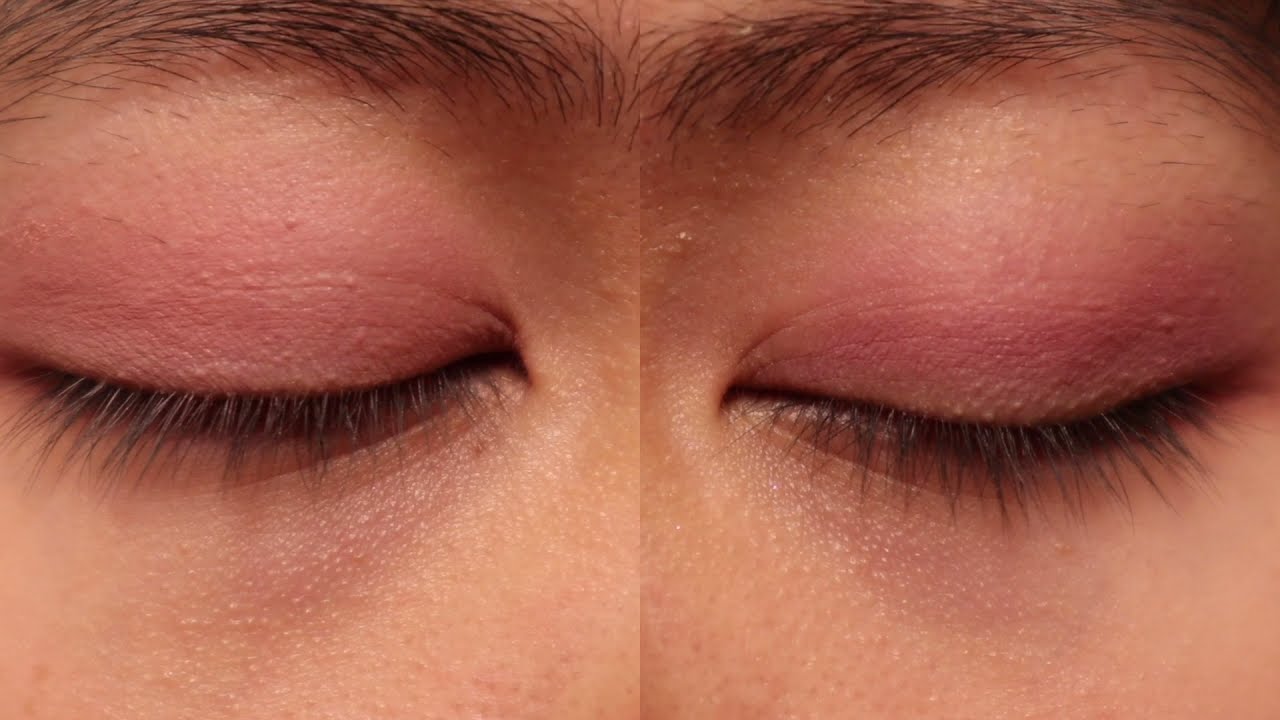The image features an extremely close-up shot of two closed eyes that appear juxtaposed, almost merging but not entirely seamless. Both eyes belong to a light-skinned individual. On the left side, the eye has dark, well-defined brows and long, dark brown eyelashes. The eyelid shows a hint of lighter pink color, possibly eye shadow. On the right side, the eye also has full dark brows but seems slightly less dense, as if partially plucked. The eyelashes are dark and straight, and the eyelid has a darker pink hue, possibly makeup. The split in the image suggests two separate photographs placed side by side, creating a mirrored yet fragmented appearance. Visible pores accentuate the high resolution of the close-up, capturing fine details such as texture and slight variations in skin color around the eyes.